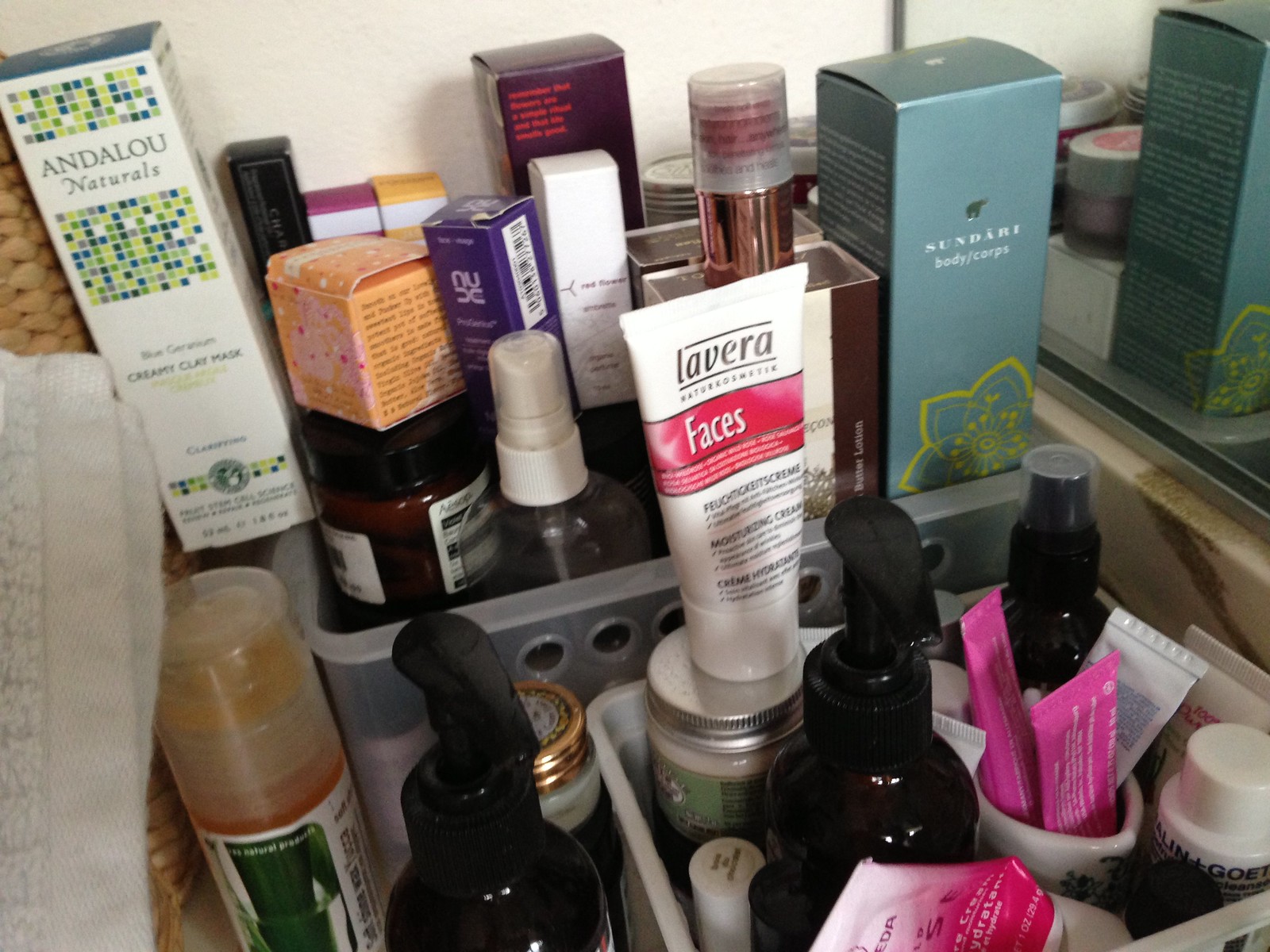This photograph, oriented in landscape mode, provides a close-up view of an array of toiletry products, meticulously organized within two baskets. The clear outer basket, adorned with small circles along its rim, holds a variety of colorful items. Nestled in front is a smaller white basket, also brimming with assorted products. On the top left, a white box from Andalou Naturals features a vibrant pattern of blue, green, and yellow. Toward the bottom center, two sleek black bottles stand prominently. Just behind them, a white tube marked with "Libera" and "Faces" in a red stripe is noticeable. The composition also includes a light blue box at the top right, along with other boxes and tubes showcasing hues of pink, brown, green, and purple, creating a vibrant and organized display.